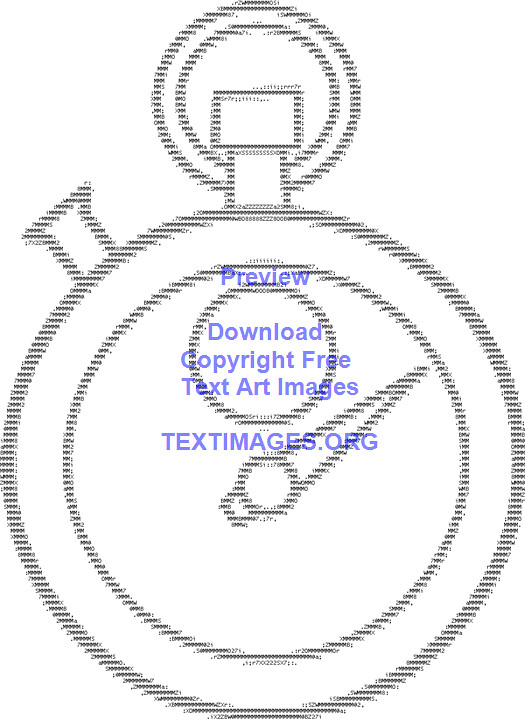This image is a computer-generated graphic of a classic round stopwatch, resembling 19th and early 20th-century timepieces. The stopwatch is centrally positioned on a white background, with black stenciling forming its outline. On closer inspection, the lines of the stopwatch are composed of intricate rows of numbers and letters, creating a serrated, textured appearance. There are distinctive features like stems at the top and upper left, likely used for winding or setting the watch, and a circle at the top for attaching a chain. The central face of the stopwatch displays a smaller inner circle bordered with black dots, with a dial pointing to 2 o’clock. Superimposed over the entire image in a purple-blue text are the words: "Preview, Download Copyright-Free Text Art Images," followed by "textimages.org" underneath. This design is indicative of the text art generated from the website textimages.org.